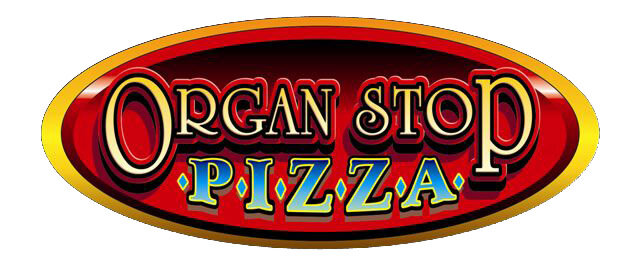The logo for Organstop Pizza, featured in an elongated horizontal oval, presents a vibrant and visually appealing design. The oval has a bright gold outline, which darkens towards the bottom, framing a rich red interior background. The name "Organstop" is prominently displayed in slightly larger yellow, 3D capital letters that seem to be elevated against the red background. Below it, the word "PIZZA" is written in capital blue letters, each character separated by small blue diamonds and outlined in yellow, adding a lively touch. The dual tones of red within the oval enhance the overall richness of the design, making it a standout sign likely adorning the front of the establishment.